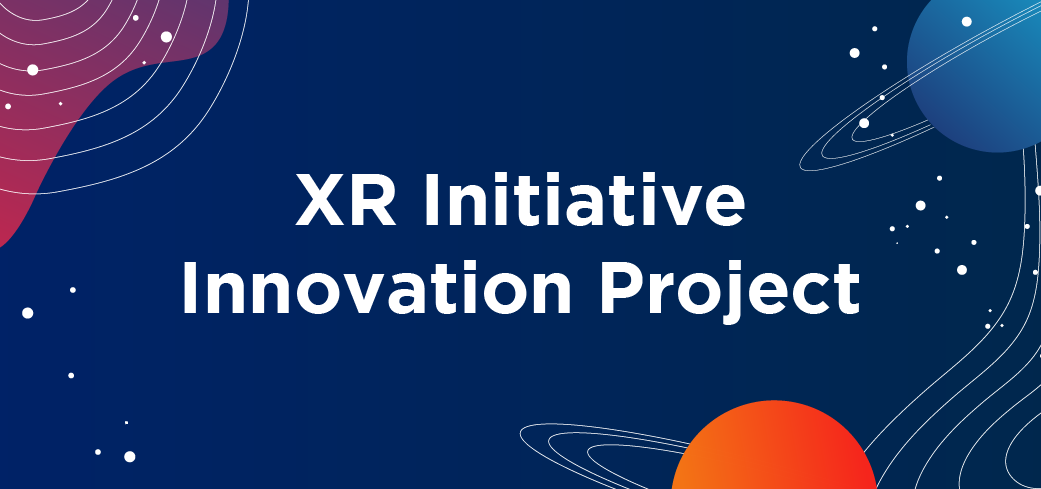The digital graphic features a horizontally rectangular image with a predominantly blue background. In the center, large white block text reads "XR Initiative Innovation Project." In the upper right corner, there is a stylized blue planet adorned with white rings and surrounded by white dots, which resemble stars or moons. Directly below this, in the lower right corner, is a bright orange planet also encircled by white rings. In the lower left corner, scattered white dots are visible, while the upper left corner showcases a red area with a series of white circular lines, resembling ripples, emanating from outside the frame and interspersed with white dots. The absence of a border gives the image an open, expansive feel, further accentuated by the dispersed elements.